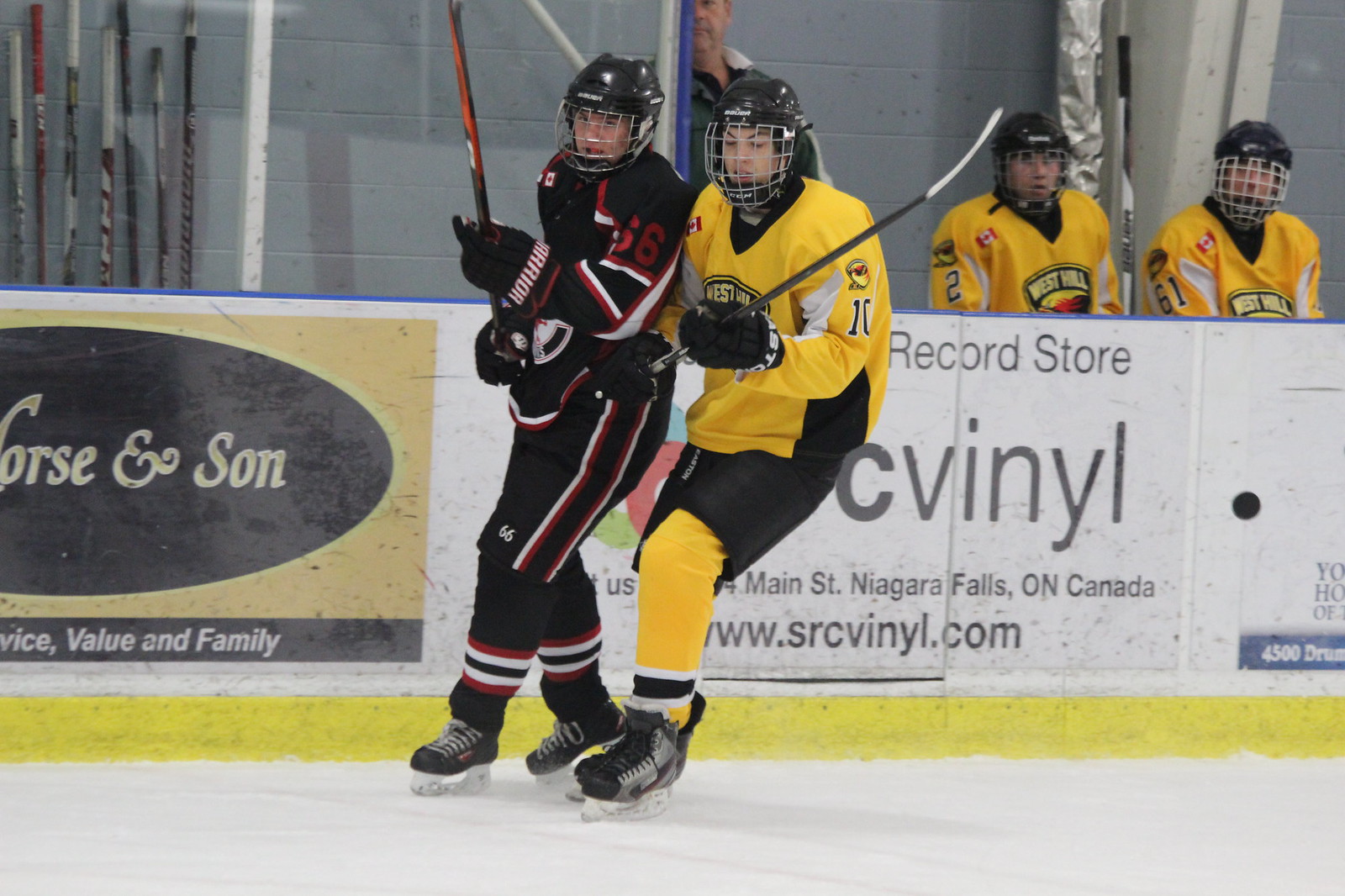In this photographic image set indoors at a hockey arena, two hockey players glide on the ice, their sticks raised. One player wears a black jersey with red and blue stripes, while the other is dressed in yellow with black pants, marked as number 10. Nearby on the right, two seated teammates in yellow jerseys with black helmets, numbers 2 and 1, watch the action closely. To their left stands an older man in a blue shirt, possibly the coach. The gray wall in the background displays several advertisements: one partially reads "O-R-S-E company" and "V-I-C-E service," another emphasizes "value and family," and a third advertises a record store with the text "srcvinyl.com, Main Street, Niagara Falls, Ontario." To the left side of the image, a few hockey sticks lean against the wall, completing the busy scene within the arena.